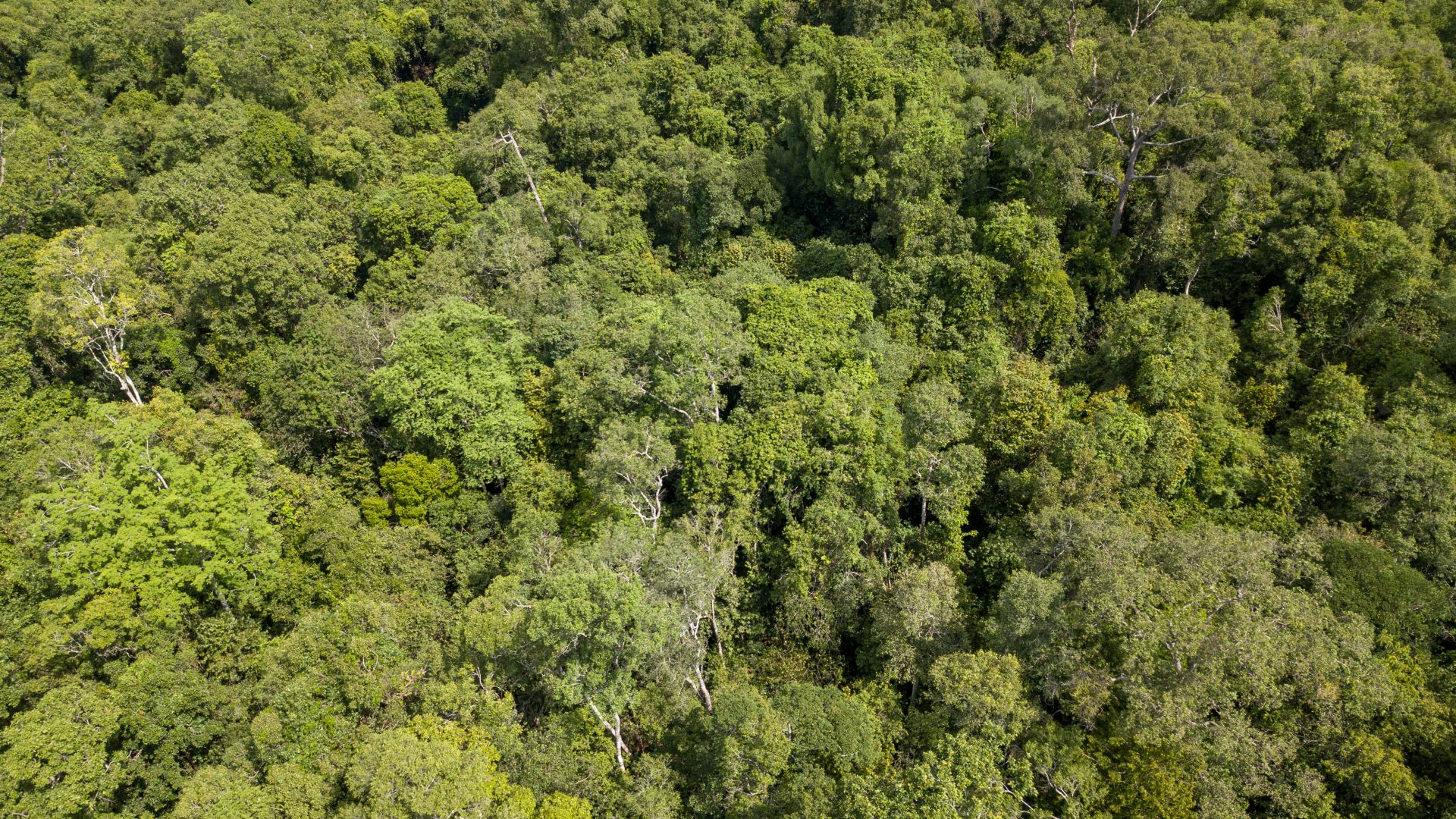This aerial, bird's-eye view captures a dense and expansive forest, showcasing a stunningly lush canopy of medium to dark green treetops. The forest is so thick that no ground is visible beneath the verdant foliage. Scattered throughout, especially towards the left-hand center and right-hand areas, a few thin white tree trunks rise slightly above the green expanse, adding texture to the scene. In the upper right quadrant of the image, the density of the trees thins out just a bit, though it’s still filled with greenery. Overall, this vibrant, green vista highlights the natural beauty and vastness of the forest.